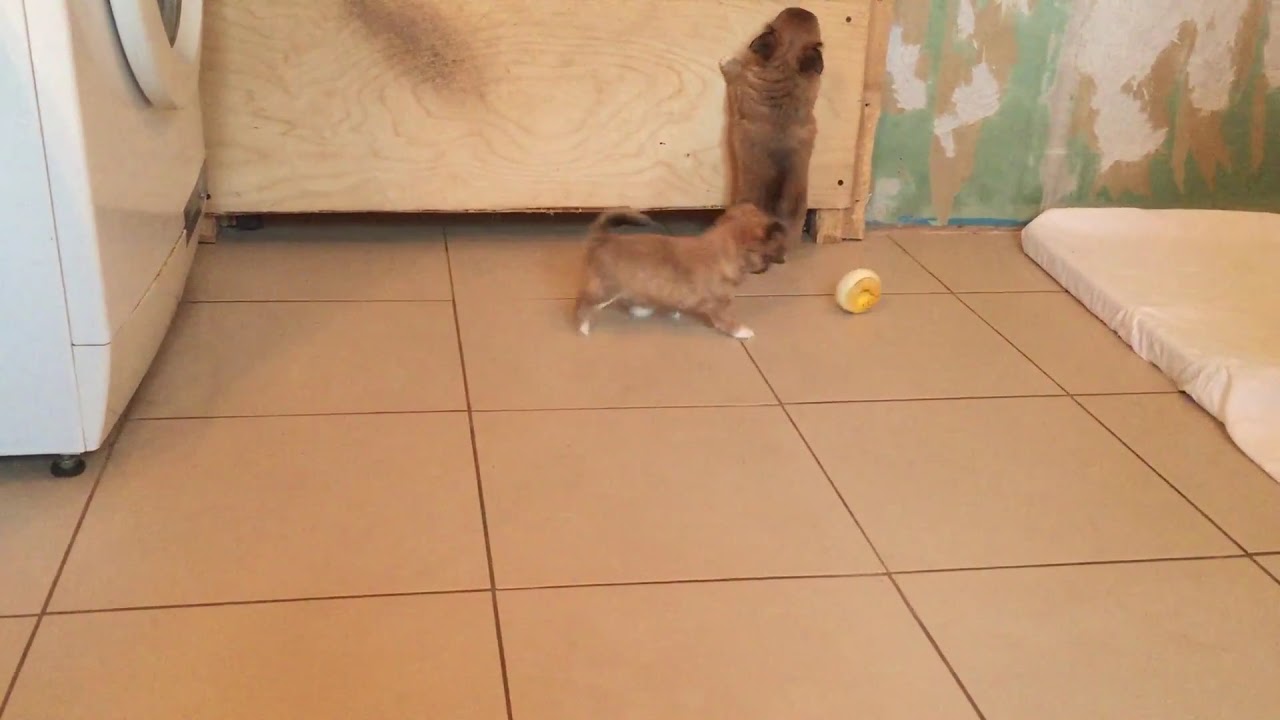This full-color horizontal photograph depicts an indoor scene featuring two playful puppies on a light brown tiled floor. In the left part of the image, there is a white, front-loading clothes dryer with a circular door. A wooden board has been erected against a wall behind the puppies, partially painted in white, green, and brown. On the right side of the photograph, there is a small white mattress lying on the floor, potentially serving as either a doggy bed or a pee pad. One puppy, a dark brown dog with black streaks and ears, seems to be trying to climb up the wooden board. Meanwhile, the other puppy, a small brown dog with white paws, is chasing a little yellow ball, which looks somewhat like a donut, in the foreground. The overall setting suggests a lively and domestic environment likely situated in Asia.